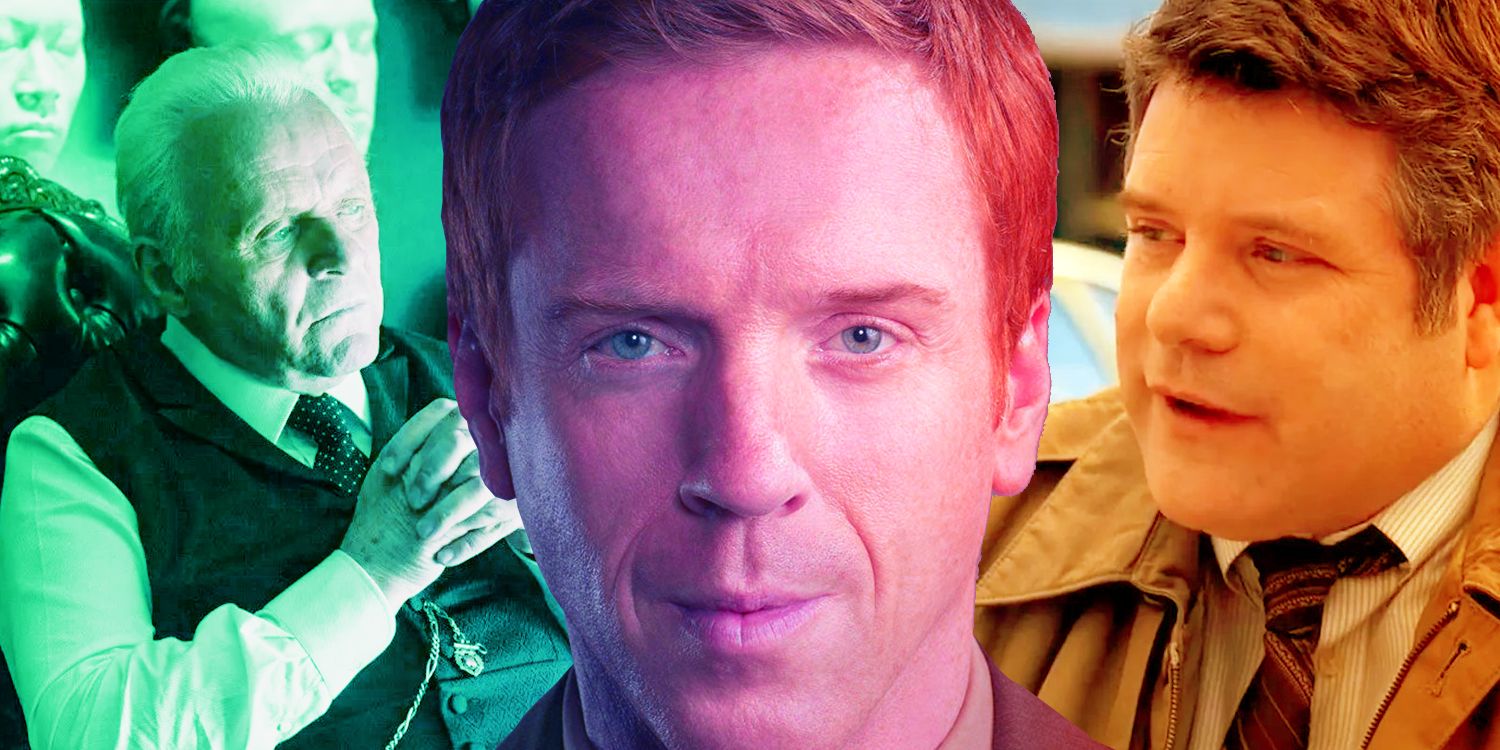The image depicts three distinct men, each captured with different lighting effects. On the left is Anthony Hopkins, known for his portrayal of Hannibal Lecter, sitting in a leather-bound chair. He has white hair, is dressed in a black suit vest and a white button-up shirt, and is wearing a white and black polka dot tie. The lighting on his image casts a light green tint, adding to the atmospheric feel. 

In the center, there's a close-up shot of a man's face from the neck up with a strong pinkish-purple lighting effect. His blue eyes and detailed facial features are prominent due to the extreme zoom and dramatic lighting.

On the right, Sean Astin is depicted wearing a brown suit jacket over a button-up pin-striped shirt paired with a red and black striped tie. His image has a normal color tone, and he is looking towards the center of the photo, contrasting sharply with the green tint of the image on the left and the pink hue of the central figure. The overall setting of the image is bright and clear, emphasizing the unique lighting and detailed expressions in each section.